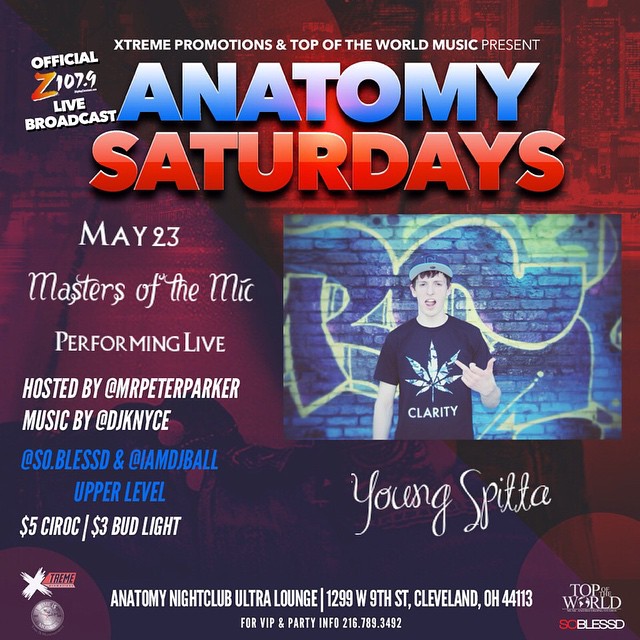This vibrant advertisement poster announces a live performance event titled "Anatomy Saturdays" with a rich blend of colors and vivid text details. The poster's background is a gradient mix of reddish-brown, purple, and red hues. At the very top, it reads "Extreme Promotions and Top of the World Music Present" in white letters, followed by the main event title: "Anatomy Saturdays," where "Anatomy" is highlighted in large blue letters and "Saturdays" in equally large red letters. 

On the left upper corner, it states "Official Live Broadcast" in white text, supplemented with "Z107.9" signaling the broadcast station. Scattered across the left side are details for the event: the date "May 23rd", and the event "Masters of the Mic Performing Live." It mentions notable hosts and performers, including "@Mr. Peter Parker," and music by "@DJ KNYCE," "@so.blessed," and "@I_am_DJ_Bol". Additionally, it notes admission fees as "$5 for Upper Level" and "$3 for Bud Light."

The right side of the poster showcases a photograph of a performer standing against a blue graffiti-adorned wall. The performer is attired in a black t-shirt featuring a marijuana leaf graphic and the word "Clarity" beneath it. He also dons a blue knit cap, contributing to his street-style aesthetic. Beneath the image, the text reads "Young Spitta," identifying the performer in the photograph.

At the very bottom of the poster, further text and logos are present, including affiliations and sponsors. The bottom left and bottom right corners are populated with logos, while the lower text gives essential logistical details like the name and address of the nightclub hosting the event.